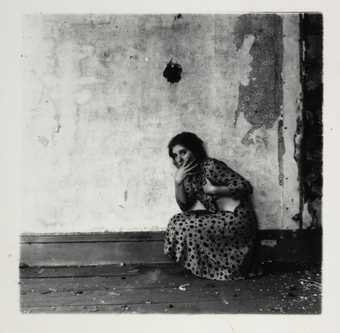This image depicts an old, black-and-white photograph of a woman in a deteriorating room. The photo is grainy and slightly out of focus, conveying a sense of age and neglect. The woman, with long dark hair, is dressed in a long dress that appears to have a floral or polka-dotted pattern, although the specifics are unclear due to the black-and-white nature of the image. She is squatted down against a large, tarnished white wall, her pose conveying distress as she rests her head in one hand and covers her mouth with the other. The room appears to be in a state of serious disrepair; the wooden plank floor is littered with debris, possibly from the crumbling wall or other sources. The wall behind her is marked with dark smudges and areas where the paint has peeled away, further emphasizing the dilapidated condition of the space. The overall atmosphere of the photograph suggests abandonment and desolation, capturing a poignant moment of apparent anxiety or contemplation.